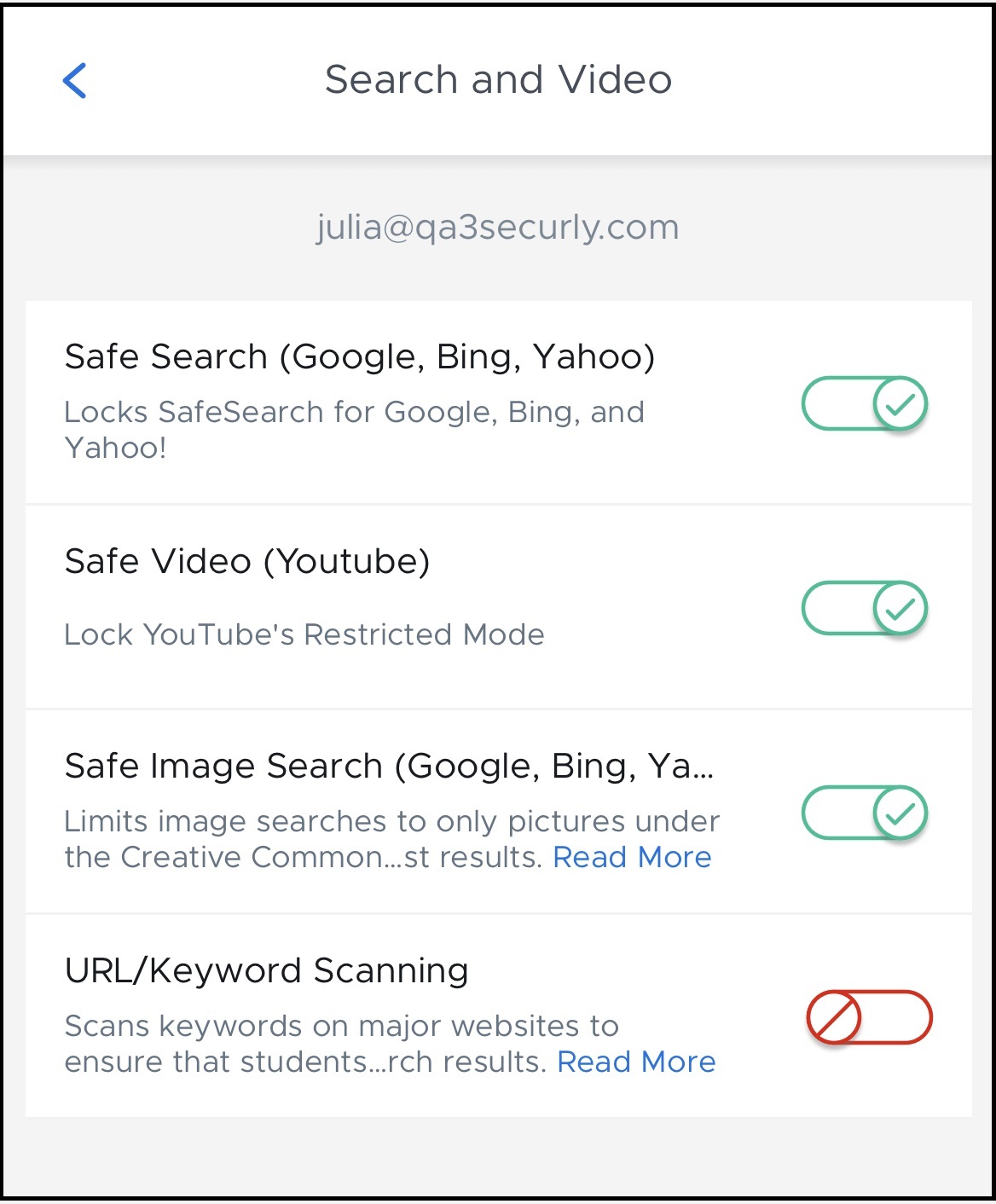This screenshot captures the settings page of an application, characterized by a clean and functional layout. At the top of the screen, there is a prominent white bar centered with the text "Search in video" displayed in dark grey or black font. To the left of this text, there is a blue back arrow button for navigation. Below the search bar, a grey section displays the email "Julia@QA3Securely.com."

The main content area features a list of toggle settings, each accompanied by a description and an associated toggle switch located on the right side. The settings include:

1. **Safe Search** (Google, Bing, Yahoo): This setting is toggled on, as indicated by a green Google checkmark.
2. **Safe Video** (YouTube): This setting is also toggled on with a similar green Google checkmark.
3. **Safe Image Search** (Google, Bing, Yahoo...): Enabled with a green Google checkmark.
4. **URL Keyword Scanning**: This final setting is toggled off, identified by a red circle with a diagonal slash (a "do not" symbol).

The boundaries of the image are defined by a thin black border, further emphasizing its structure.